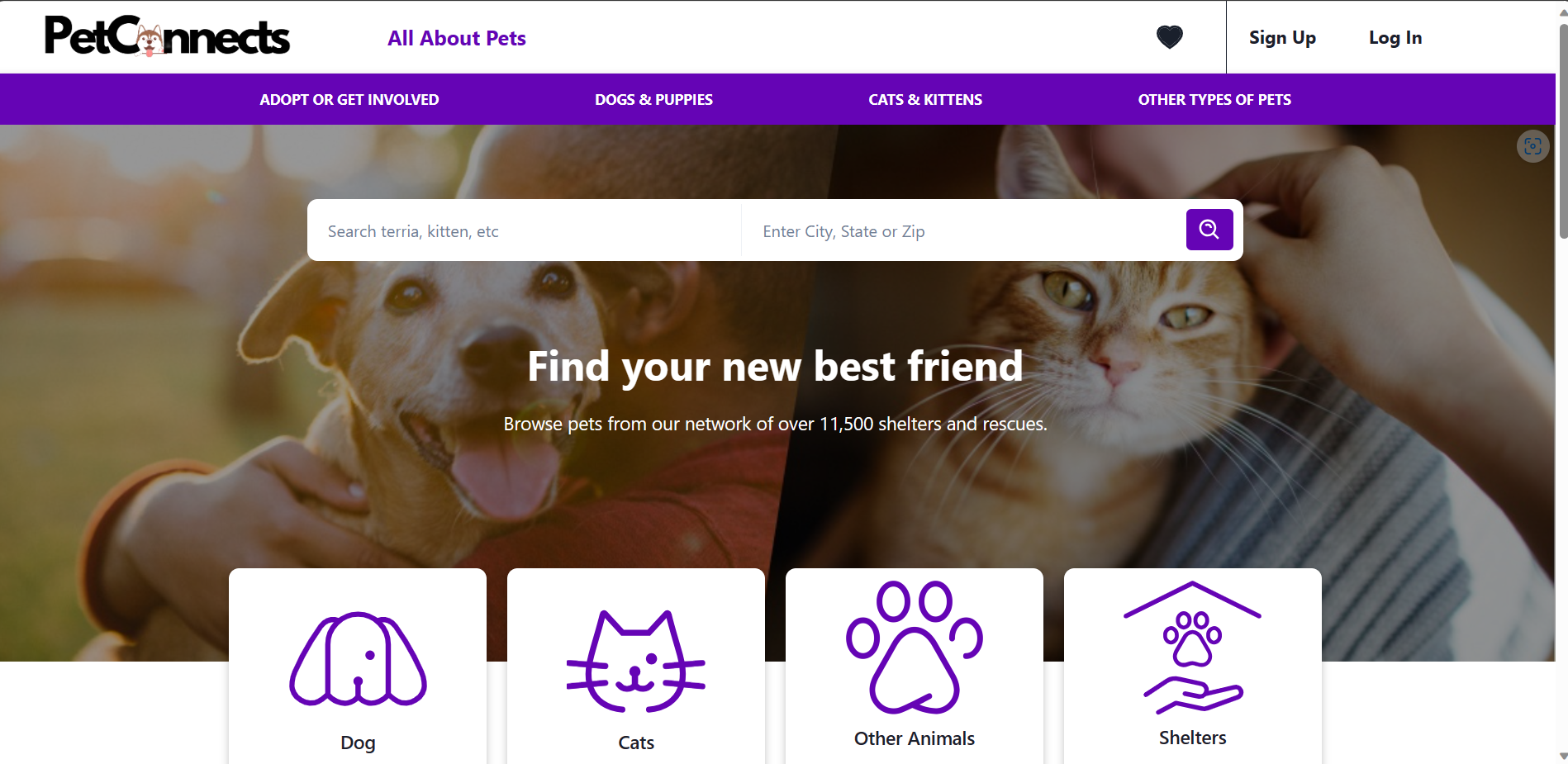PetConnex Website for Animal Adoption

At the top of the PetConnex homepage, a sleek white navigation bar spans the width of the page. On the far left, "PetConnex" is prominently displayed in black font, with the "P" and "C" capitalized. Ingeniously, the "O" in "Connex" is replaced with a charming illustration of a brown husky head, complete with its tongue playfully sticking out. Adjacent to this logo, "All About Pets" is elegantly written in purple font. On the far right, the header features a grey heart icon followed by "Sign Up" and "Log In" options.

Beneath the navigation bar, a bold purple strip presents critical options in white text: "Adopt or Get Involved," "Dogs and Puppies," "Cats and Kittens," and "Other Types of Pets." A search bar is conveniently placed here, allowing users to look for specific pets by entering keywords, city, state, or zip code.

Just below the purple strip, the text "Find Your New Best Friend" invites users to explore pets from over 11,500 shelters and rescues. This message is also in white font, clearly standing out against the backdrop. The background features a heartwarming image: a dark-skinned man holding a light brown dog with an open mouth and a long, happy tongue, and another person—whose gender is indistinct—cuddling a reddish cat with orange-yellow eyes and subtle stripes.

At the bottom, four icons in purple on a white background categorize the types of animals and facilities: the first icon labeled "Dogs" shows a dog, the second, labeled "Cats," displays a cat, the third labeled "Other Animals," features a generic paw, and the fourth, labeled "Shelters," portrays a paw inside a hand beneath a roof, symbolizing protection and care.